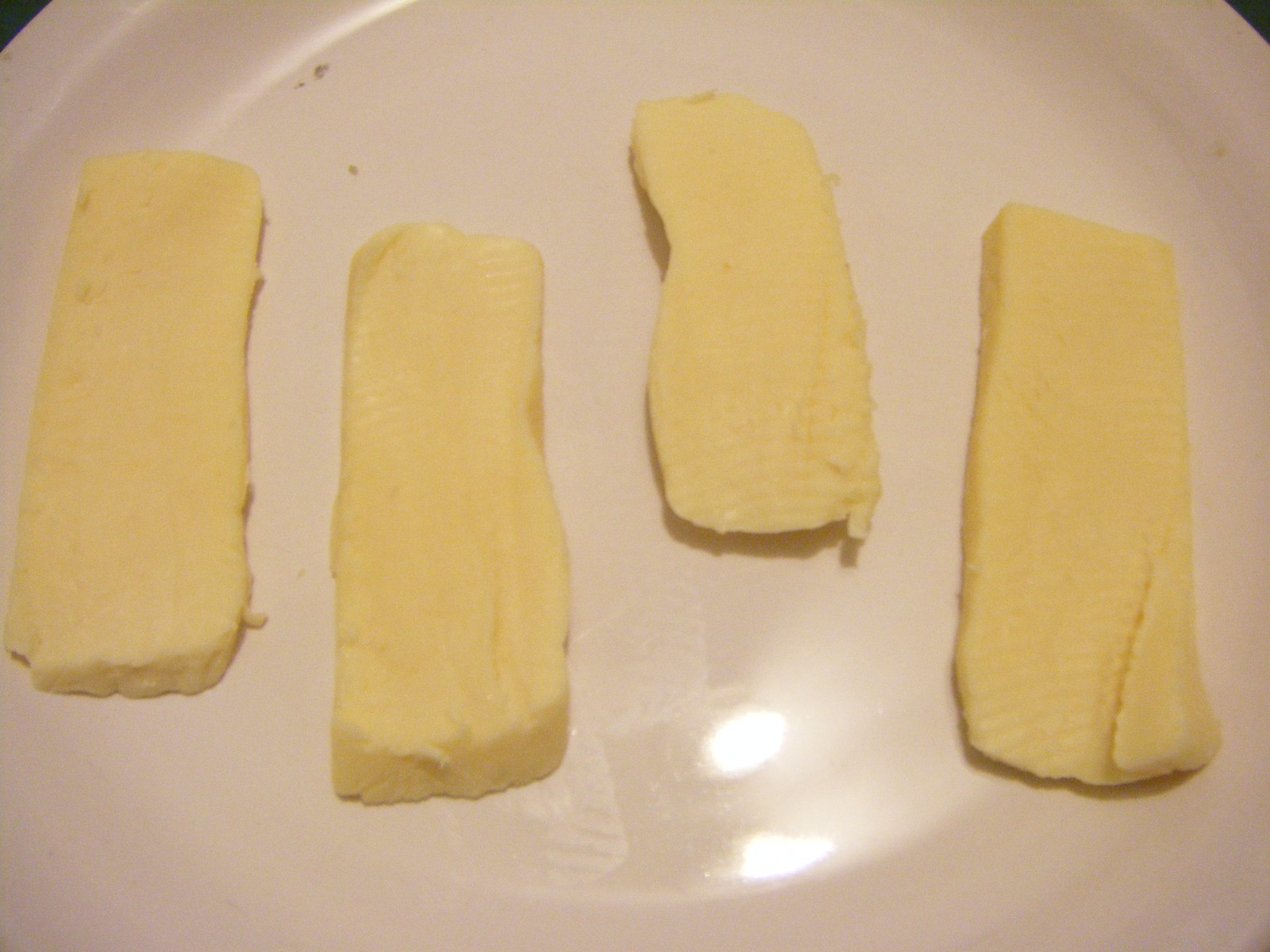This close-up photograph captures a white, circular glass plate sitting atop what appears to be a black surface, possibly a table. Upon this plate, which is reflecting bright overhead light, are four rectangular-shaped pats of butter. These pats of butter, pale and light yellow in color, have been cut lengthwise from a stick of butter. The cuts have left striations and ridges across the top surfaces, indicating they were made with a butter knife. The pieces are arranged in an artful but asymmetrical manner: one pat sits in the left center, with another slightly below it, one slightly above, and the fourth positioned similarly to the second. Despite the effort to arrange the butter artfully, the plate has small gray and black specks of dirt, detracting from the overall presentation.